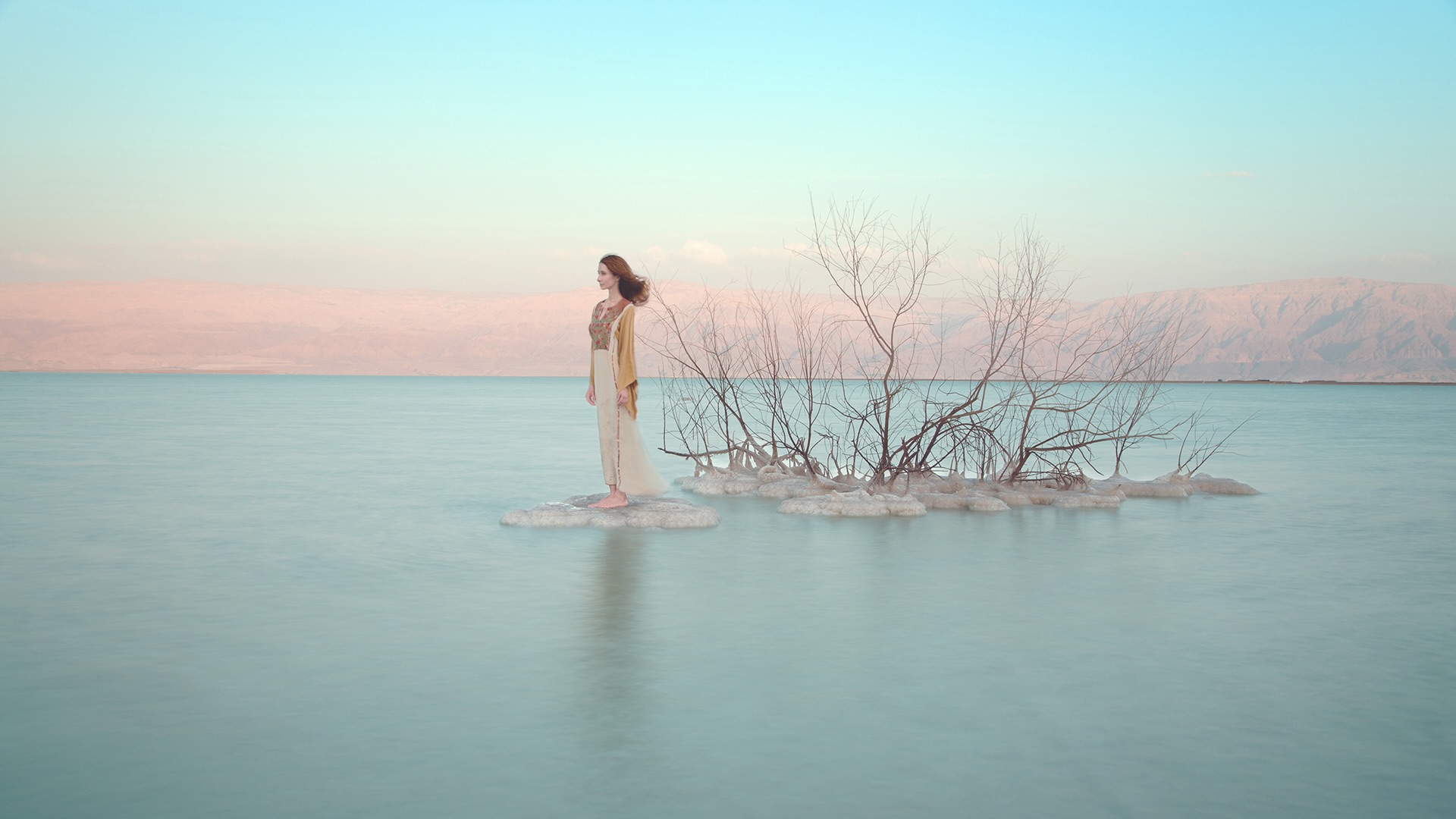A woman stands serenely on a small, rocky islet in the middle of a tranquil lake. The water is a smooth, light greenish-blue with barely noticeable ripples, mirroring a faint reflection of the woman. She is dressed in flowing, earth-toned attire: a cream-colored, long skirt matched with a golden, wide-sleeved top. Behind her, another larger set of rocks juts out, adorned with scraggly, leafless bushes and dead trees, adding a touch of starkness to the scene. The sky above transitions from a deep blue to a soft pink hue near the horizon, devoid of clouds but subtly gloomy, casting a calm, muted light over the lake. In the distant background, snow-capped mountains rise majestically, completing the picturesque and ethereal landscape. Brown-haired and barefoot, the woman exudes a sense of peaceful isolation in this natural tableau.